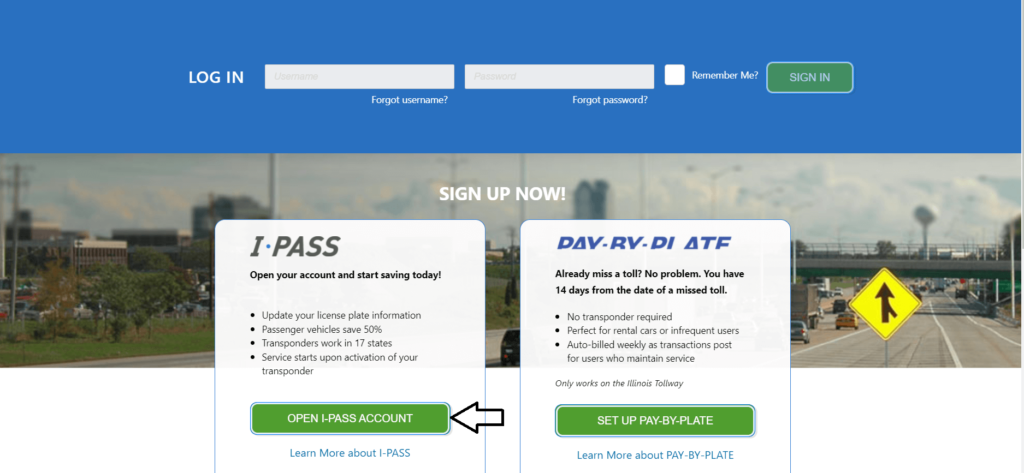The screenshot is a rectangular image of a website interface, with its top and bottom sides longer than the left and right sides. At the top of the screenshot, a blue banner spans from the top left to the top right corner. Centrally positioned within the banner, slightly towards the left, is white text that reads "Login," followed by a white rectangle to enter a username and another white rectangle below it to enter a password. Beneath the username entry field is a white text link that reads "Forgot Username" while beneath the password entry field, white text reads "Forgot Password."

To the right of the password entry box is an unchecked white square checkbox labeled "Remember Me" in white text. Further to the right is a green rectangle with a white border, featuring white text in the center that reads "Sign In."

The main backdrop of the image is a photograph of a bustling highway scene. On the left side of this background, there are multiple two- to three-story industrial or commercial buildings. On the right side, there's a multi-lane highway with traffic moving in both directions, accompanied by both pedestrian and vehicle overpasses.

Overlaid on this highway background are two white rectangles with multiple lines of text. The text in the left rectangle reads: "I-PASS: Open your account and start saving today. Update license plate information. Passenger vehicles save 50%."